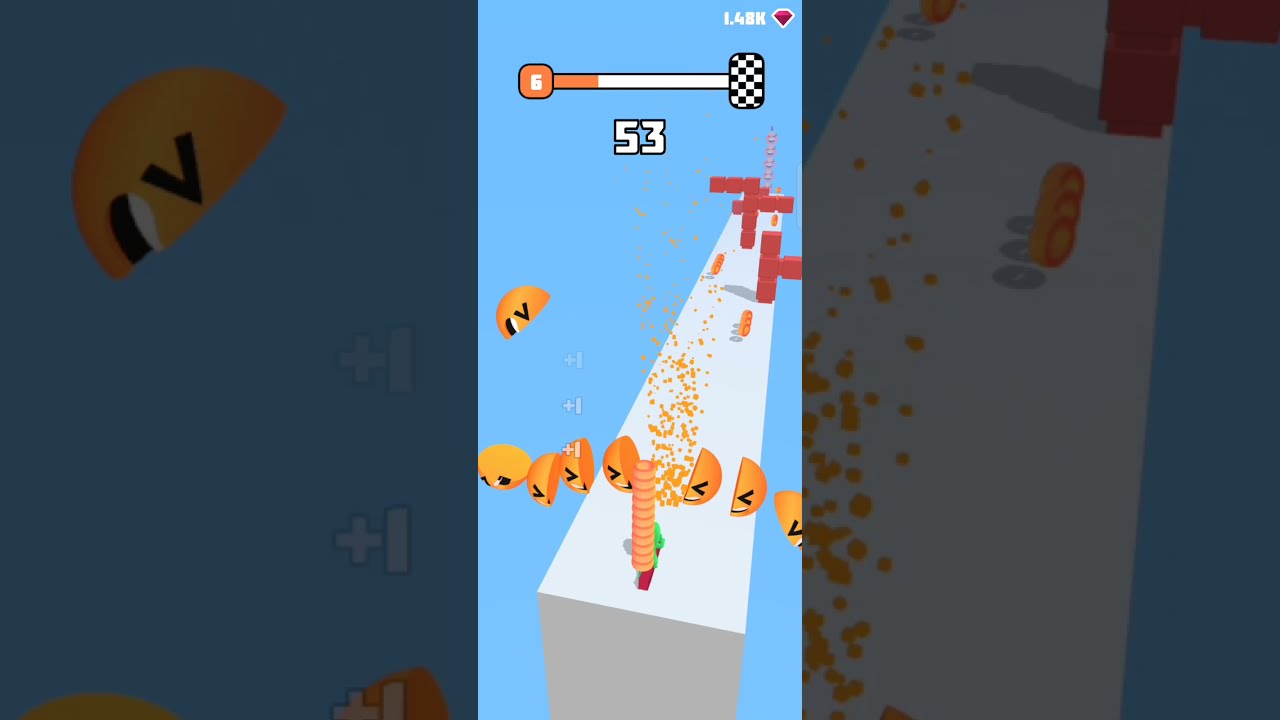The image features a light blue background, with a central white platform resembling a long table strewn with numerous elements. Scattered across this platform are semicircular orange shapes, reminiscent of Pac-Man faces, which appear to be sliced in half. Alongside these, there are yellow dots and stacked red squares, giving the impression of various game obstacles or items. At the top of the image, there is a status bar with the left side displaying the number "6" next to a thermometer-like icon, and the right side showing a checkerboard pattern, indicating the finish line. The bar itself is partially orange, suggesting a loading or progress indicator. Underneath this bar, in white numbers with a black outline, the score "53" is prominently displayed. Situated in the top right corner, a magenta gemstone icon is accompanied by the number "1.48k," possibly representing a form of in-game currency. Overall, the image depicts a mobile game interface where players seem to chop faces in half and collect points, emphasizing the game's fun and engaging nature.